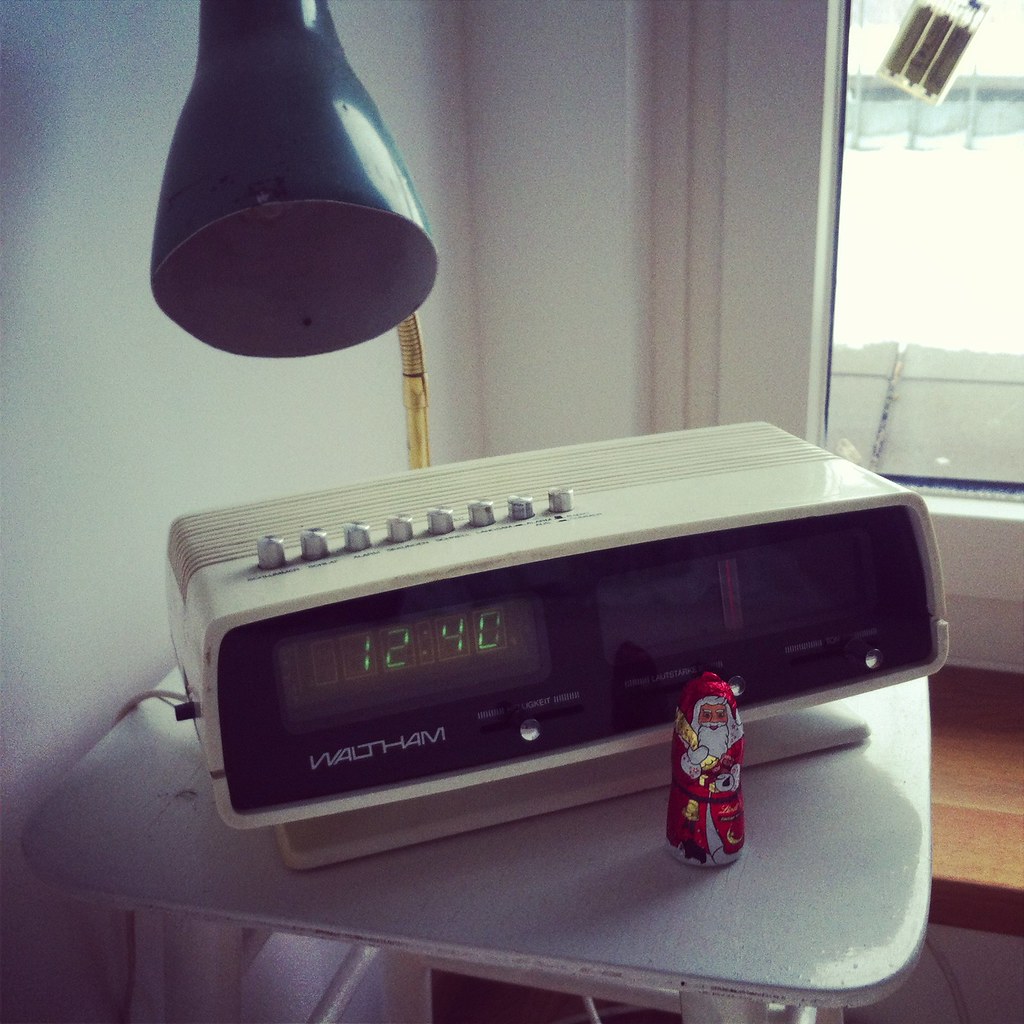In this photograph, we see the interior of a well-lit room characterized by its white walls and medium-toned wooden floors. Central to the image is a square table with rounded edges, featuring a glossy surface in either white or light gray. Placed prominently on the table is a vintage-style clock radio, made of white and black plastic materials. The clock is rectangular with rounded corners and showcases a black face with green LCD digits displaying the time as 12:40. The brand name "Waltham" is inscribed in white on its surface. In front of the clock radio stands a small foil-wrapped chocolate in the shape of Santa Claus, enhancing the festive feel of the scene. Positioned behind the clock is a stylish desk lamp with a brass arm and a conical, blue shade, adding a touch of elegance to the room.